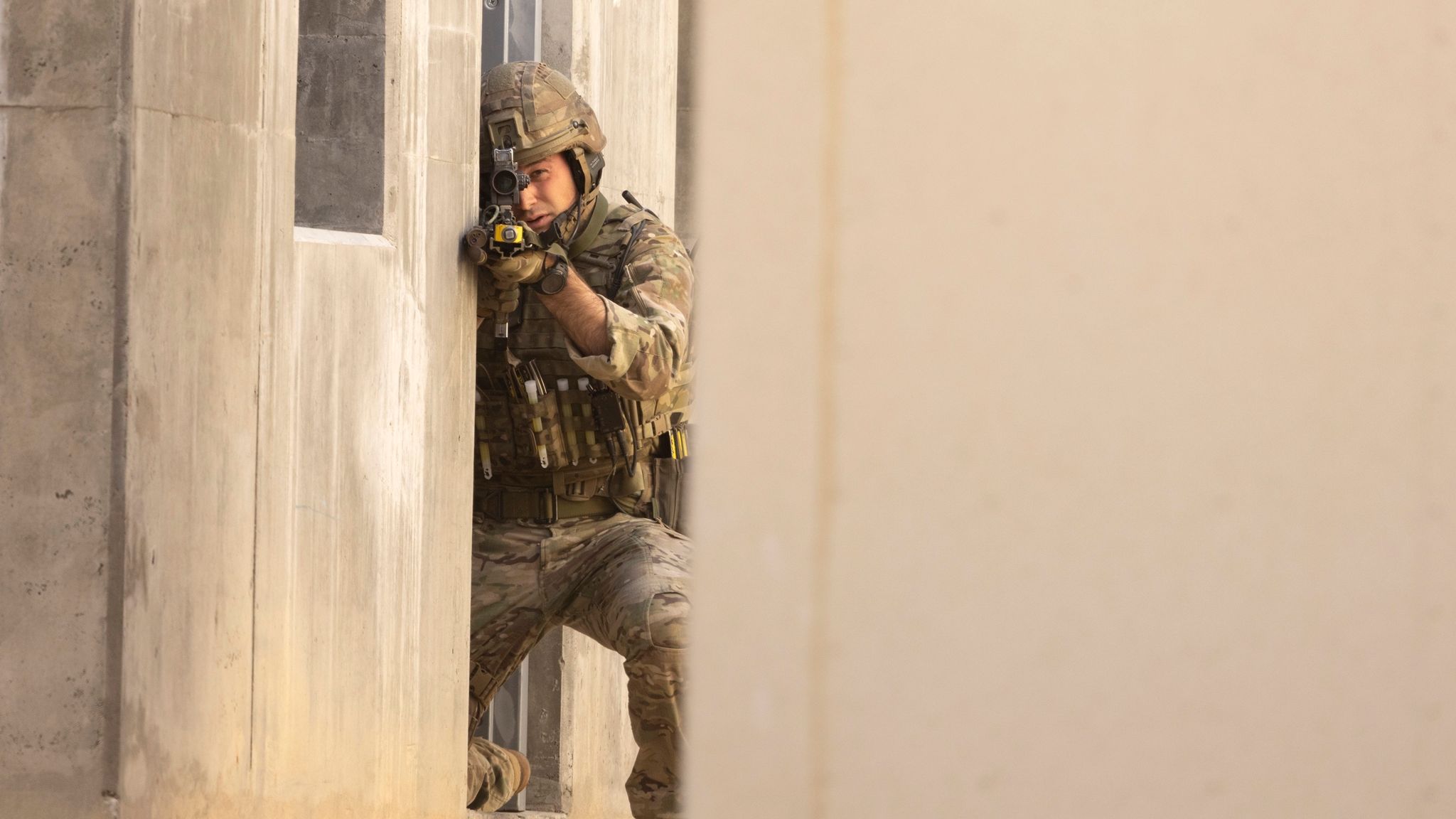In this striking photograph, a soldier clad in full military combat gear—including a tan-colored desert camouflage uniform, tactical vest, helmet, and gloves—is captured in a tense moment. Equipped with a utility belt and bearing numerous straps filled with various objects, the soldier kneels on one knee, steadies himself, and peers through the sight of a rifle directly at the camera. Only half of his face is visible, revealing his left eye, nose, and mouth, with the rest obscured by the firearm. The soldier is positioned slightly off-center to the left, taking cover in the concrete nook of a building with weathered, light brown cement walls that show streaks from exposure to the elements. The scene vividly conveys a high-stakes combat situation, emphasizing the soldier's focused gaze and the stark urban environment surrounding him.